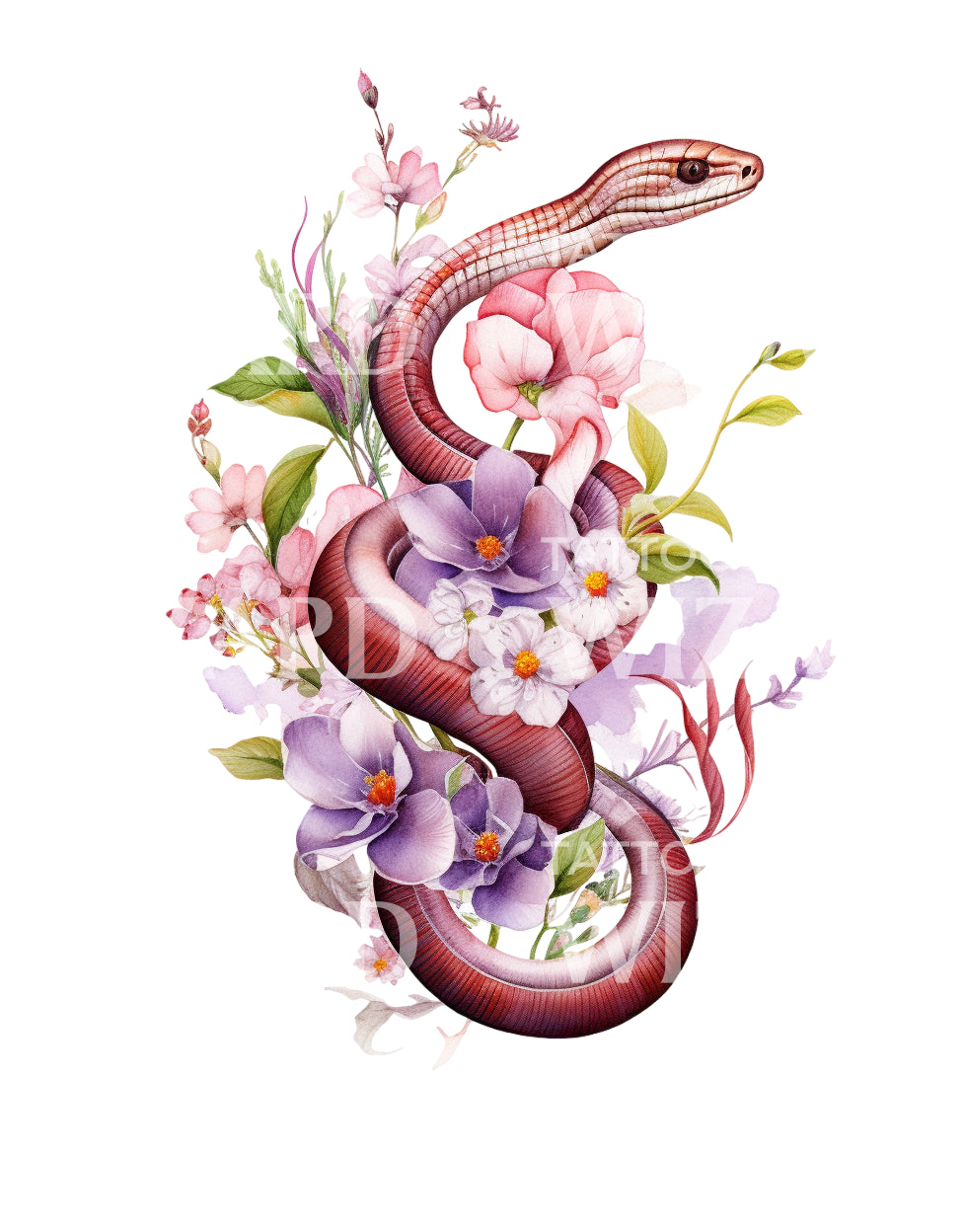This detailed illustration depicts a vibrant red snake, transitioning to pink along its belly, coiled gracefully around an ornate arrangement of flowers and foliage. The snake, adorned with distinct, square-shaped scales, has mesmerizing red eyes. Intertwined with green leaves, the bouquet features a variety of flowers, including prominent purple lilies, delicate pink roses, and other white and pink flowers nestled between the snake’s coils. The drawing showcases the snake slithering upwards with a lifelike quality, yet clearly delineates it as an illustration. Subtle lettering, spelling out "T-A-T-T-O" twice, can be discerned within the artwork, adding an intriguing layer to the piece.